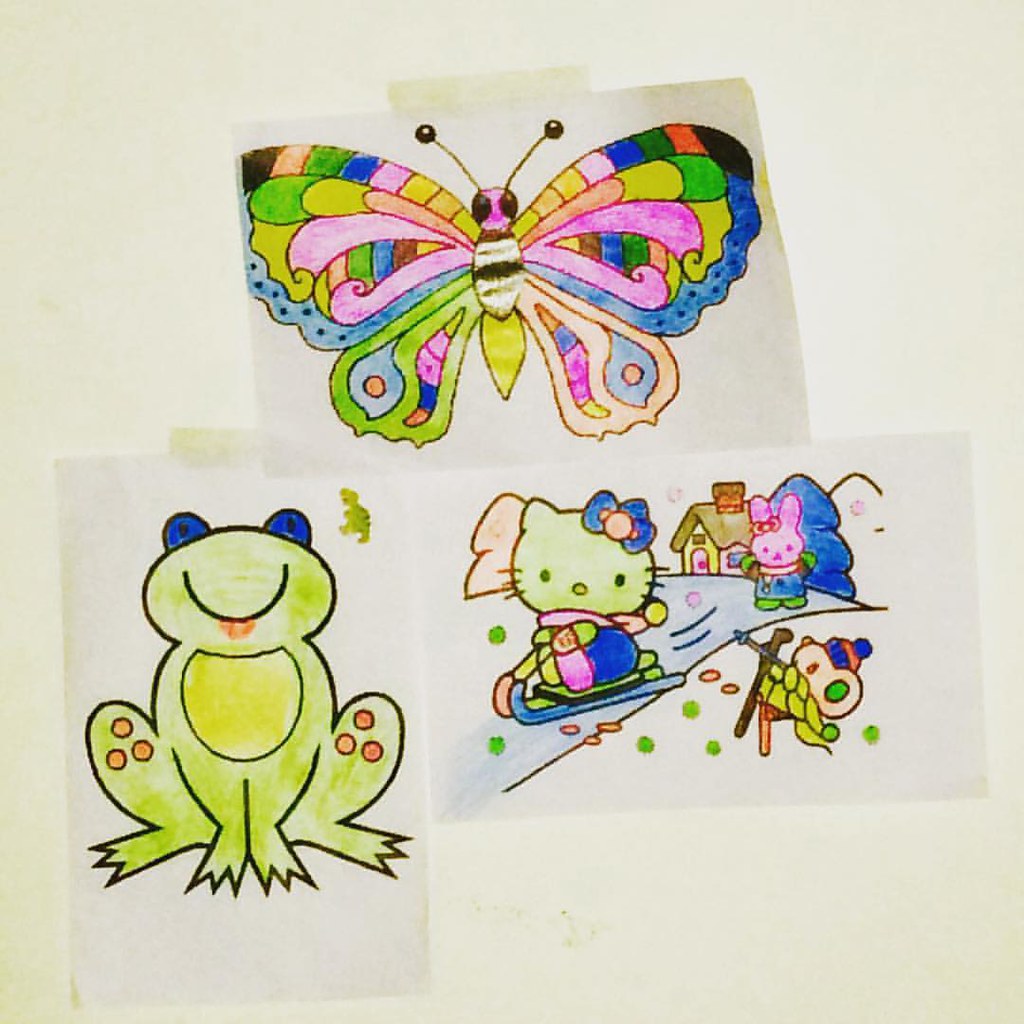This photo captures three carefully colored drawings, likely created by a child of around seven years or older, and taped to a white surface, such as a wall or fridge, with tape visible at the bottom of each picture. 

1. The top drawing is a vibrant butterfly in landscape format. It features a rainbow of colors, including green, pink, light blue, orange, dark blue, yellow, light orange, black, and brown. The butterfly's head is pink, and it has black eyes and yellow antenna with black circles on the ends. The wings showcase a complex pattern with a black outline and segments in various hues such as peach, green, blue, yellow, orange, and pink. The thorax is decorated with black and white stripes, ending in yellow.

2. The bottom left drawing depicts a frog, also in landscape format. The frog has blue eyes, an orange tongue, a yellow chest, and a predominantly green body. Notably, it has three red/orange spots on each knee.

3. The bottom right drawing portrays a Hello Kitty character sledding down a snowy hill, again in landscape format. Hello Kitty is styled with a white head tinged with yellow and is dressed in a dark blue shirt and pink scarf. She rides a lime green sled with different colored blades—one peach and the other dark blue. Accompanying characters include a peach-colored mouse wearing a dark blue hat with a red stripe, and a pink bunny with a red bow and green gloves and boots. This winter scene is set against a backdrop of blue and white trees, a small house with a brown roof, and a pink door, alongside scattered green and orange spherical objects resembling snowflakes or balls. Additionally, a character resembling a monkey appears on the right side, seemingly falling with skis on.